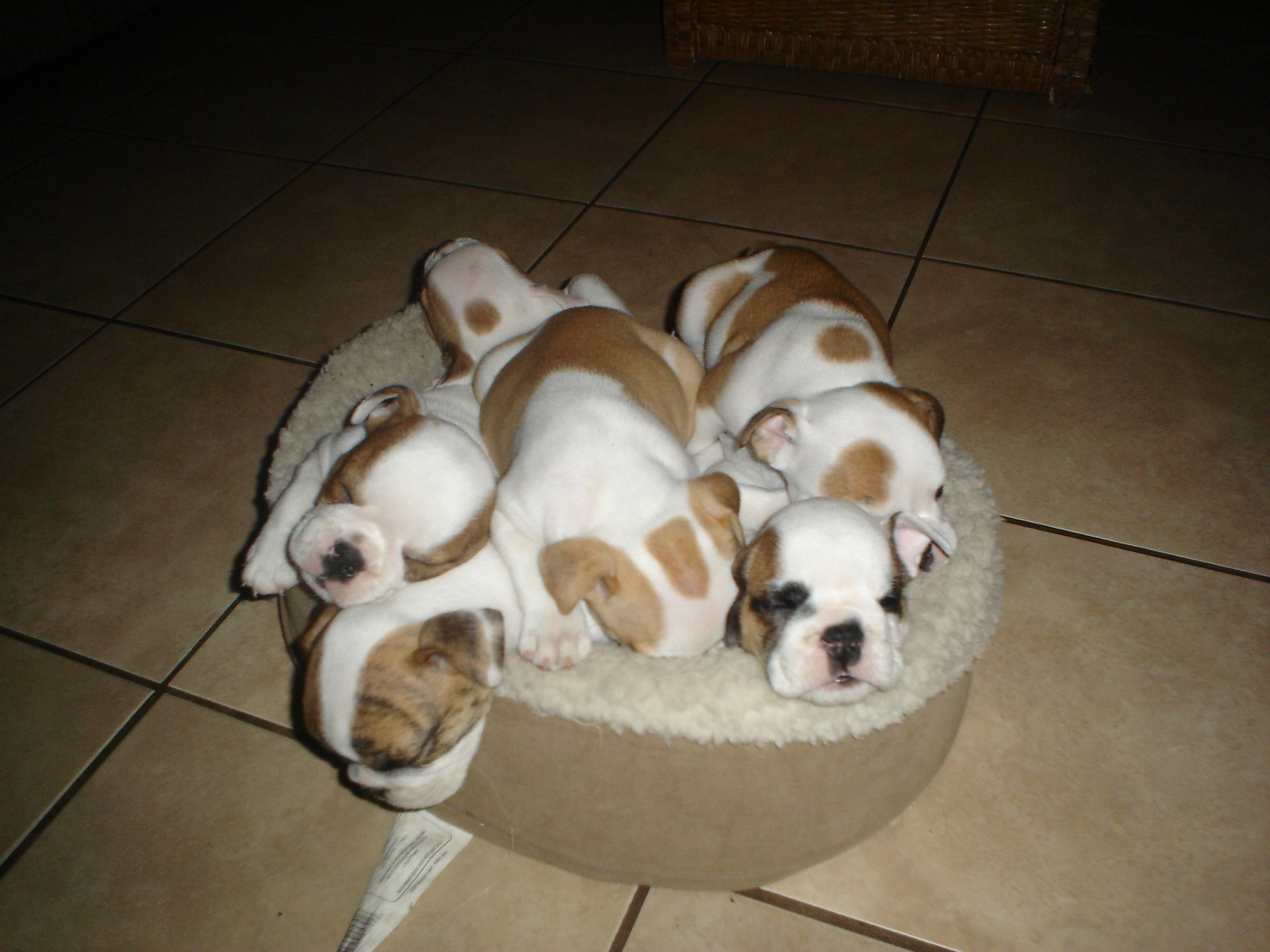The photograph captures a litter of six adorable Boxer-like puppies nestled together in a small, circular, beige puppy bed with fluffy, sheep’s wool-like lining. The puppies are crammed adorably on top of one another in the cozy bed, which is centered on a light brown tile floor with black grout lines in a dramatically lit setting. The pups have large, short-snouted heads and floppy ears, mostly white with various brown spots on their ears, around their eyes, or along their backs. One puppy's head is hanging off the side of the bed, revealing brown ears and a white muzzle with a black-tipped nose. Fluffy brown and white, another puppy has a similar coloring with a pinkish nose. Despite the varied spots and patches, their coloring blends harmoniously, making them irresistibly cute as they face the camera, with their tiny black eyes and noses caught in the focused light.